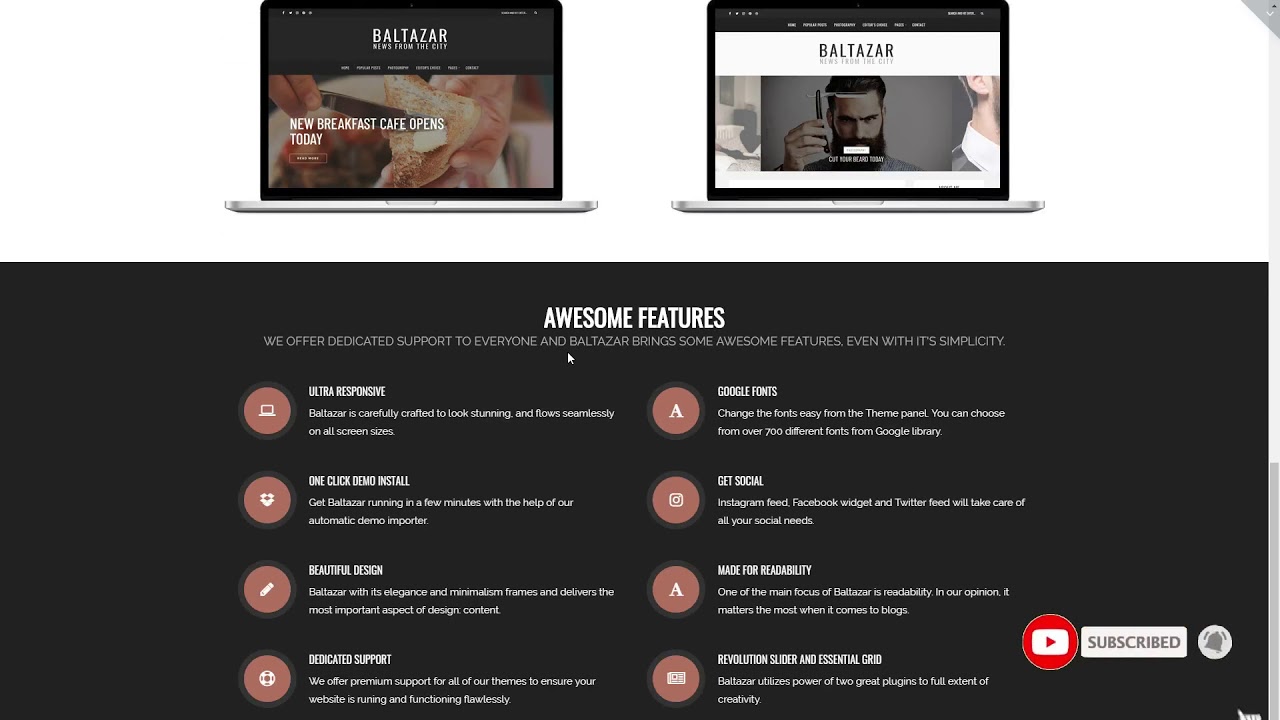The image captures two main elements promoting different offerings from Balthazar. The top section prominently features two contrasting images side by side. To the left is a darker photograph with the text "Balthazar" in white, highlighting the launch of a new breakfast cafe with a close-up shot of a hand holding a piece of buttered toast, ready to be enjoyed. On the right, there is a lighter image displaying a white banner with the word "Balthazar" in black text. Below this banner, an individual is holding what appears to be a grooming utensil, possibly showcasing the results of their personal care routine, with a neat beard trim.

Underneath these images lies a large black area with text detailing the exceptional features Balthazar offers. The description emphasizes "Awesome Features" that include ultra-responsive design, one-click demo install, beautiful design aesthetics, dedicated support, Google Fonts integration, and social media connectivity. Additionally, the platform boasts a "Revolution Slider" and an "Essential Grid", underscoring its usability for creating responsive and visually appealing websites.